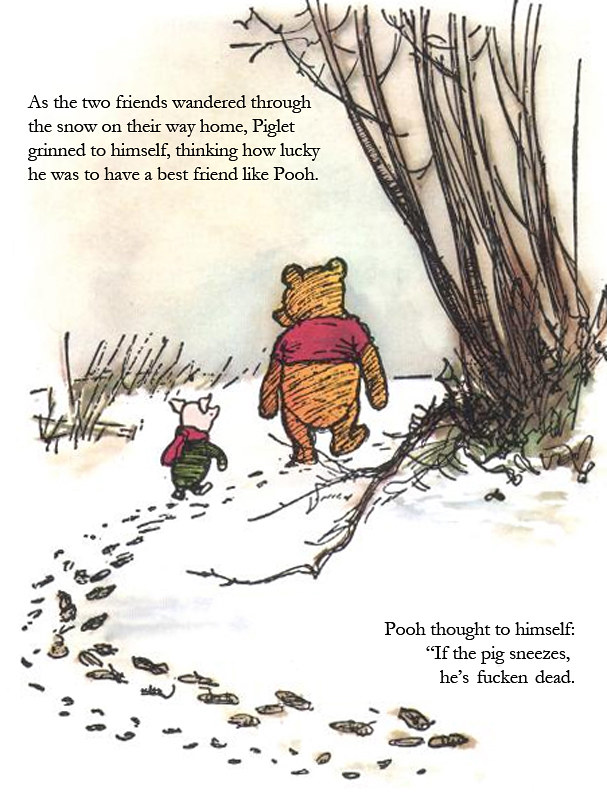This image is a cartoon illustration taken from a Winnie-the-Pooh book or comic panel, featuring Pooh and Piglet. Pooh, wearing his signature red shirt, and Piglet, adorned with a red scarf and likely a green shirt, are walking through a snowy landscape, leaving a winding trail of footprints behind them. The pair is observed from behind, with Pooh glancing over his left shoulder at Piglet. On the right side of the scene stands a bare, leafless tree, and on the left, some dying grass or weeds can be seen amid a wooden fence with metal wire. The sky above them is gray, adding to the wintry atmosphere. At the top of the image, text reads: "As the two friends wandered through the snow on their way home, Piglet grinned to himself, thinking how lucky he was to have a best friend like Pooh." At the bottom, an edited line humorously states, "Pooh thought to himself, If the pig sneezes, he's fucking dead." This added text is the only modification to the otherwise authentic book panel.